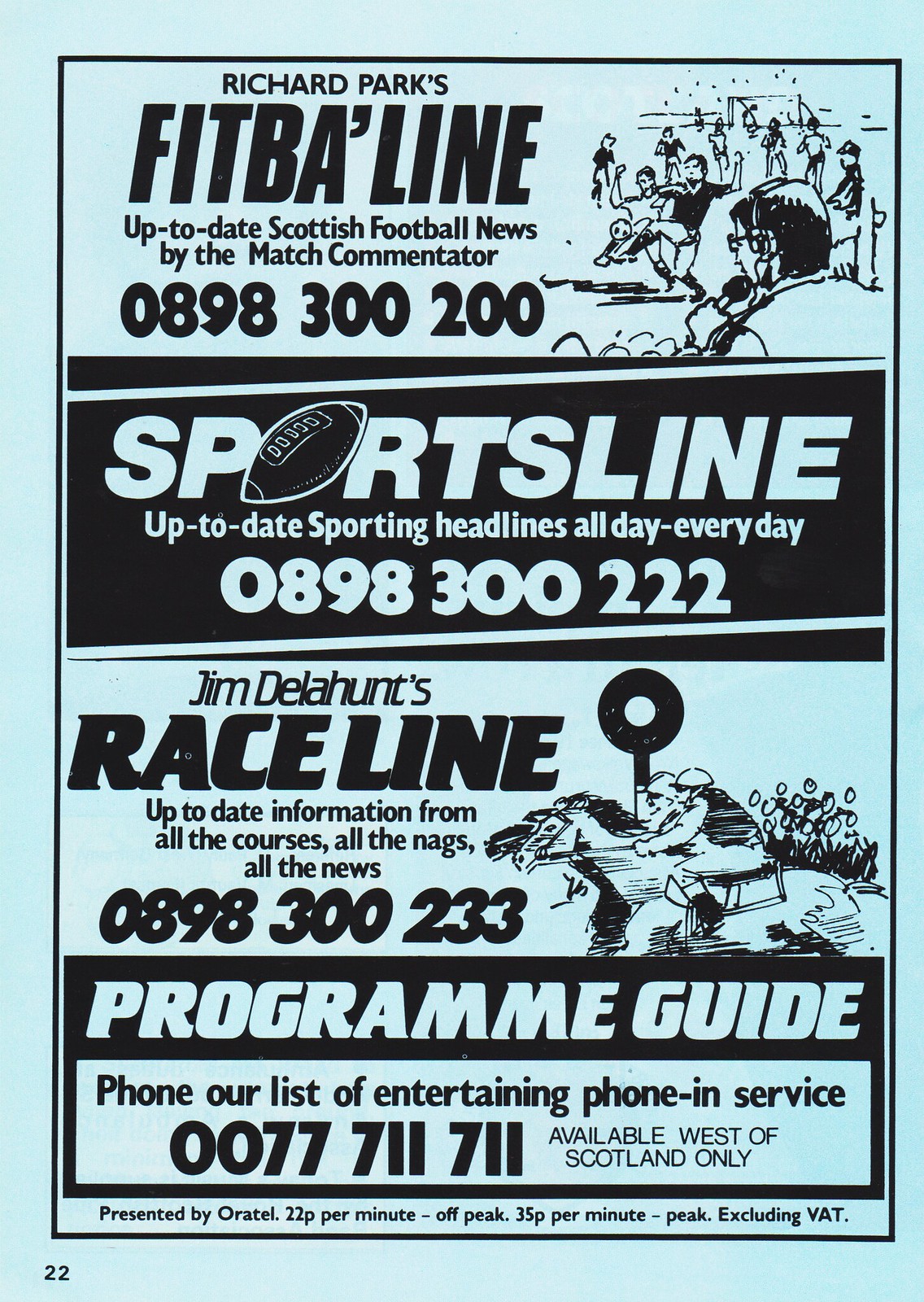The advertisement, set against a light blue background, prominently features a series of black-and-white text sections detailing various sports information services. At the top, "Richard Park's Fitba Line" offers up-to-date Scottish football news by the match commentator, with contact number 0898 300 200. Below, "Sports Line" provides up-to-date sporting headlines all day, every day, and includes a football icon in the letter "O," with contact number 0898 300 222. Further down, "Jim Delahunt's Race Line" offers comprehensive information from all the courses, detailing all the nags and all the news, with the number 0898 300 233 and a drawing of a horse race beside it. The 'Program Guide' section invites users to phone a list of entertaining services at 07771 1711, exclusive to the West of Scotland. Additionally, the advertisement notes the service provider, Oratel, with rates of 22p per minute off-peak and 35p per minute peak, excluding VAT. On the top right, there are illustrations of a crowd and an announcer holding a microphone, adding a dynamic visual element to the page, which is marked as page 22 at the bottom left.